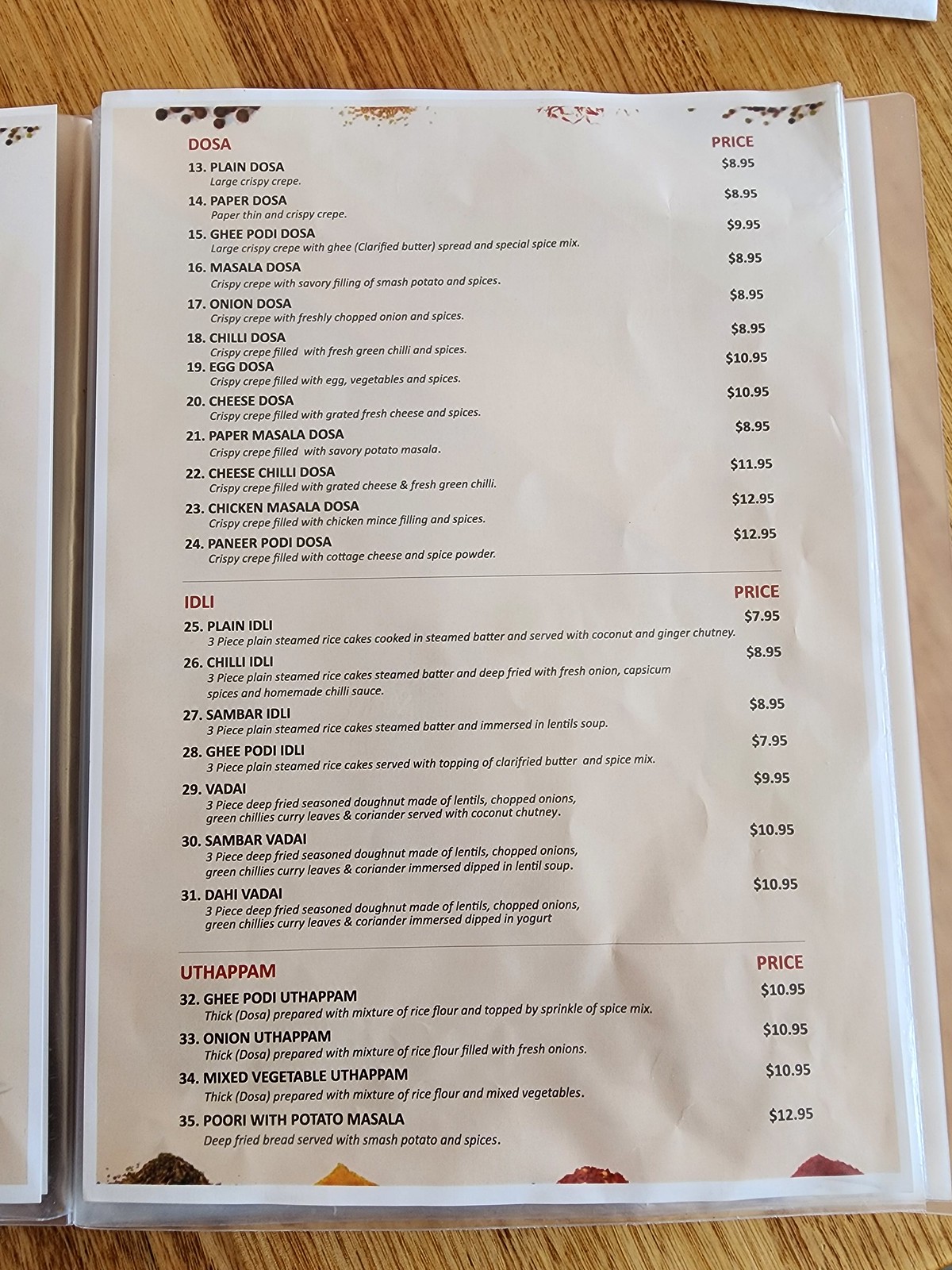This image showcases an extensive menu from an Indian restaurant. At the top of the menu, there is a diverse selection of dosas, including:

- Dosa
- Plain Dosa
- Paper Dosa
- Ghee Podi Dosa
- Masala Dosa
- Onion Dosa
- Chili Dosa
- Egg Dosa
- Cheese Dosa
- Paper Masala Dosa
- Cheese Chili Dosa
- Chicken Masala Dosa
- Paneer Podi Dosa

Following the dosa section, the menu transitions to a variety of idlis:

- Plain Idli
- Chili Idli
- Sambar Idli
- Ghee Podi Idli
- Vadai
- Sambar Vadai
- Dahai Vadai

Further down, the menu lists a selection of uttapams including:

- Ghee Podi Uttapam
- Onion Uttapam
- Mixed Vegetable Uttapam

Towards the bottom of the menu, there is an offering of Puri with Potato Masala. The layout and variety hint at a rich culinary tradition aimed at offering a broad spectrum of South Indian flavors.